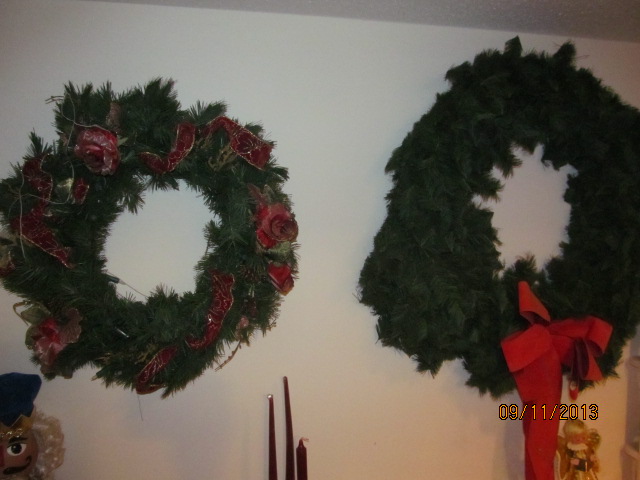This dated photograph from 09-11-2013 captures two festive Christmas wreaths hanging high on a white wall, with several other holiday decorations adding to the scene. The wreath on the left is adorned with a red and gold ribbon woven throughout, faint fairy lights, and possibly some faded red flowers. At the bottom left corner, partially visible, is the face of a nutcracker doll with blonde hair, suggesting traditional holiday decor.

The wreath on the right is larger, entirely green, and accented by a large red bow that drapes below the frame of the picture. Below these wreaths, three burgundy taper candles of varying heights stand out against the white wall, their tops just visible in the frame. Additionally, an angel figurine is positioned beneath the right wreath. In the bottom right-hand corner of the photograph, a yellow date stamp reads "09-11-2013," indicating when this festive scene was captured.